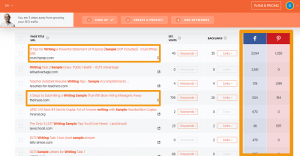The image depicts a screenshot of a web page, though it is notably blurry, making it difficult to discern the specific text and detailed content present on the page. The overall color scheme features a predominantly white background accented with shades of orange. 

At the top of the web page, there is a horizontal banner divided into two shades of orange: a darker shade on top and a more pastel shade beneath it. On the left side of this pastel orange section, a horizontal white background strip contains the outline image of a man's head and shoulders. 

The main body of the page contains several rows of text and columns, though their content is unclear due to the image's poor quality. However, two specific rows on the left side are highlighted with orange rectangular outlines, drawing attention amidst the general blur. The overall page displays a somewhat organized but indistinct structure, with the highlighted text and orange elements standing out against the white background.